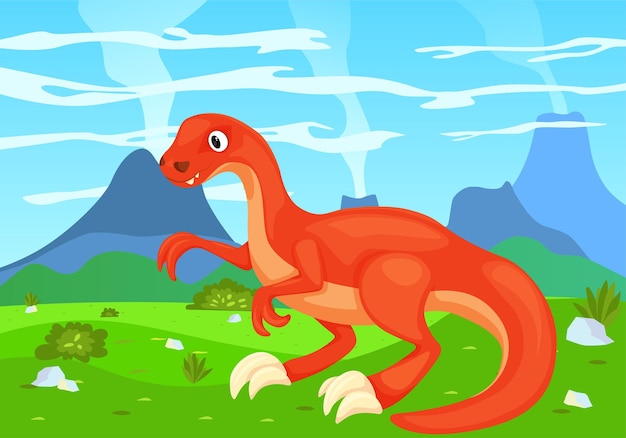The image is a vibrant, cartoonish depiction of a red dinosaur, likely a children's drawing or illustration. The dinosaur stands on green grass, characterized by its long neck, large tail, and peach-colored stomach. It has distinctive features such as two white teeth protruding from its mouth, white claws on its feet, two fingers on its hands, and three toes on its feet. The scene is set against a landscape dominated by green hills and multiple blue volcanoes, three of which appear to be erupting, with puffy white smoke billowing from them. The sky above is light blue, dotted with wispy white clouds. The foreground showcases darker green plants and some white rocks, adding to the rich detail of the image.